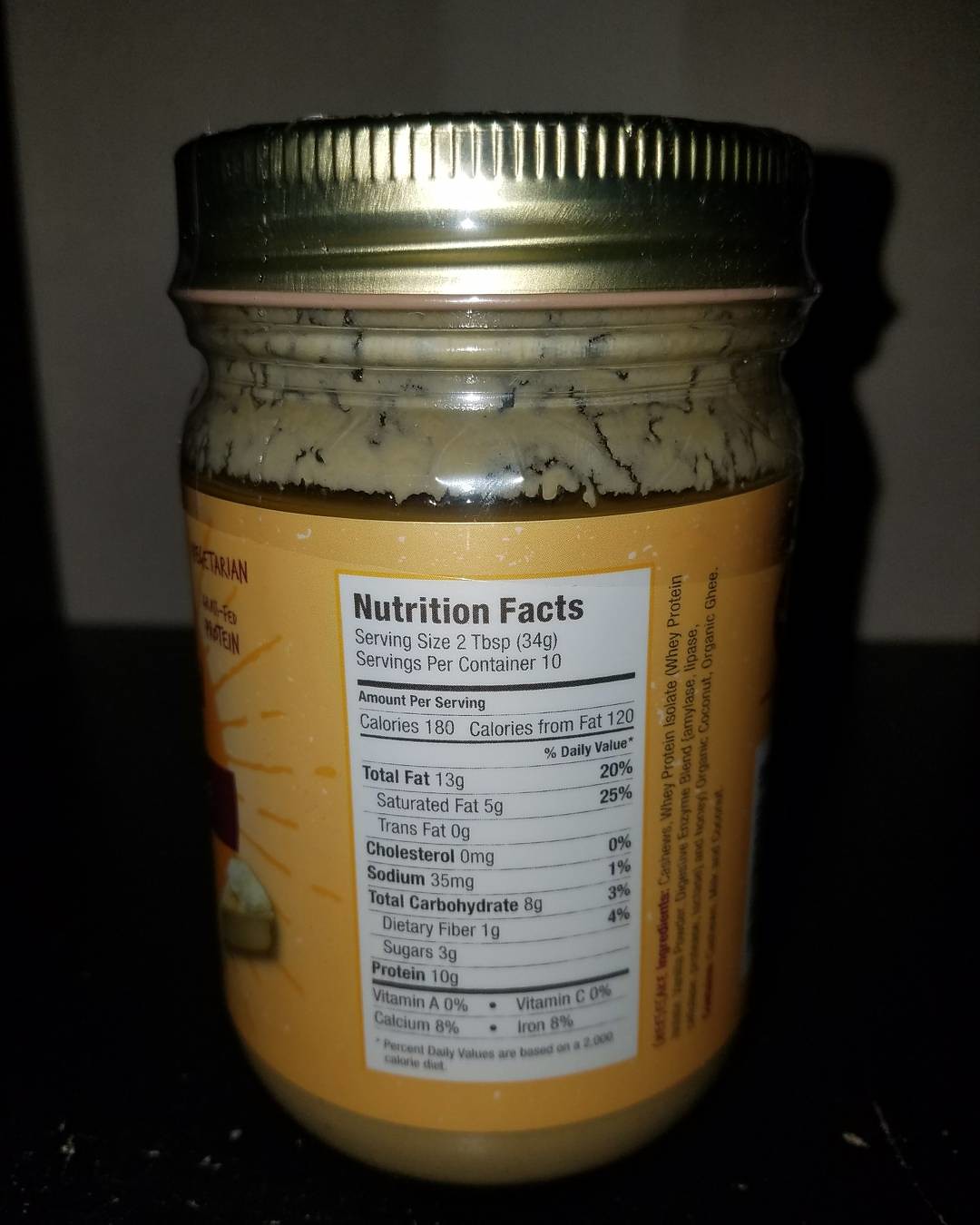This vertically oriented color photograph features a glass jar with a golden cap positioned centrally against a dark background. Prominently displayed in the center of the image is the jar's nutritional facts label, encased in a white box with bold black text. The label is affixed to an orange-colored surface, starkly contrasting with other elements of the image. Above the label, a viscous, peanut butter-like substance is notably adhered to the jar's glass surface, bridging the gap between the cap and the label. On the right side of the jar, the list of ingredients is presented vertically, though the text is too small and blurred to read clearly. To the left of the label, there is an indistinct image or graphic, adding a sense of mystery to the overall presentation. The jar sits on a dark table, casting a shadow that extends to the right, subtly touching the wall behind.